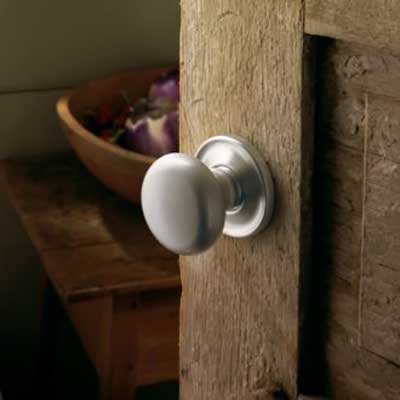The close-up image features a portion of an aged, unfinished wooden door, with a simple round silver doorknob attached to its right side. The wood appears very worn and faded, suggesting it is old and weathered, reminiscent of what might be seen in a log cabin. The door is partially open, revealing a room beyond it. To the left of the image, there is a wooden table that is somewhat shadowed, making it difficult to clearly discern. On this table, there is a wooden bowl containing violet and white flowers. The light source, potentially from a window not visible in the frame, illuminates the scene and reflects subtly off the doorknob. The overall ambiance suggests an indoor setting, with rustic and natural elements highlighted in the composition.